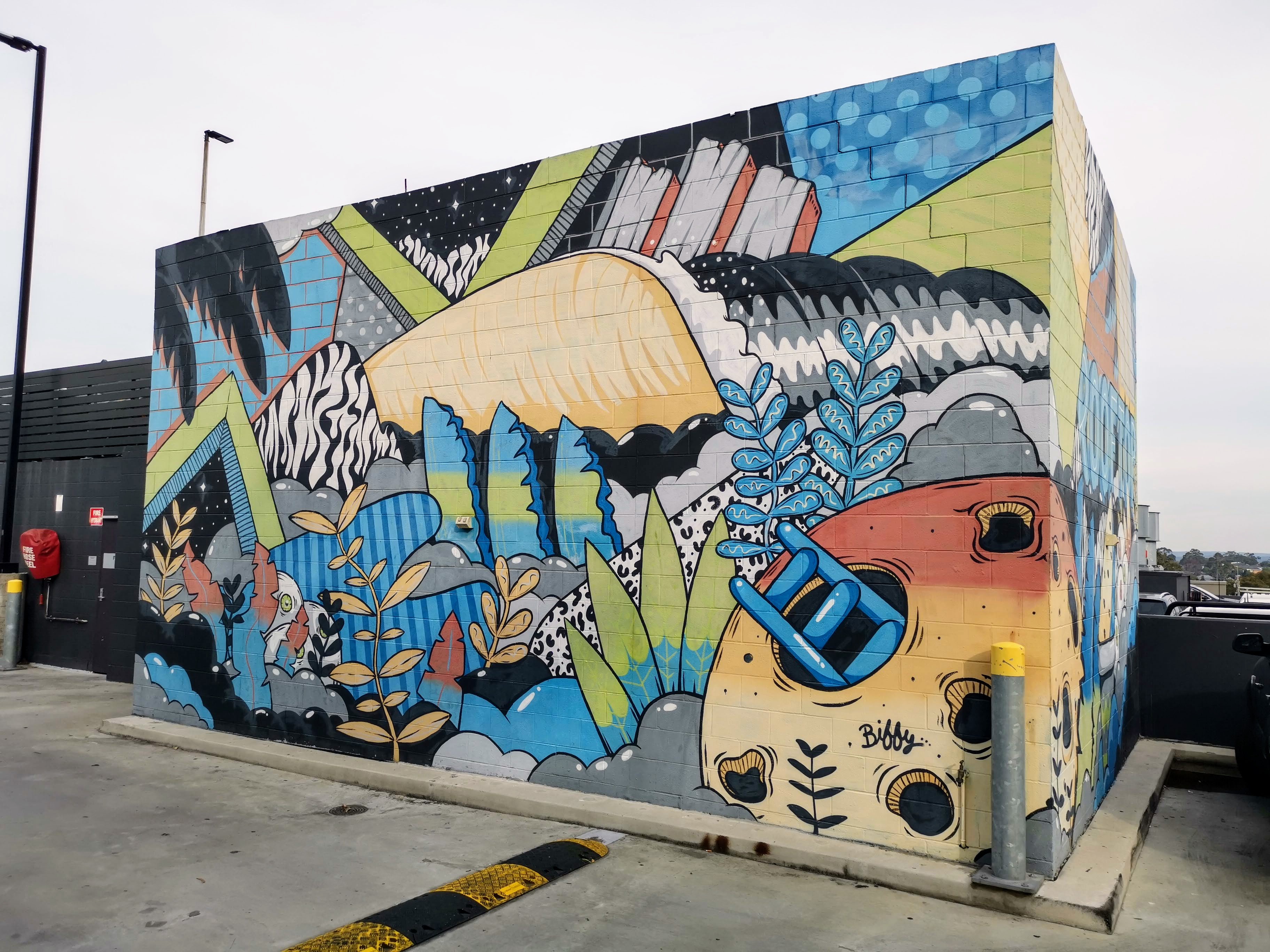This image captures a vibrant and detailed mural painted on the side of a building in what appears to be a parking lot or rooftop setting. The mural is nature-themed, showcasing a rich tapestry of colors including blues, yellows, greens, and grays. A notable feature is a moon situated at the bottom right of the composition, with a blue ladder emerging from one of its craters. Surrounding the moon are an array of leaves—green ones beside it and blue ones above. The mural also depicts wave-like patterns rendered in both gray and yellow hues.

Adding to the complexity of the scene, there is a green border with a small blue section within it. The backdrop simulates a night sky dotted with stars, and to the left, palm fronds stretch out. The setting features elements suggesting a building environment, including a black door and a stone floor, with a speed bump in front. A contrasting black building is visible to the left of the mural, and to the right, there are trees and parked cars, indicating it may be a restaurant or drive-thru area. The word "Dilly" is prominently displayed on the mural, and several black dots are sprayed artfully across the surface, enhancing the professional, street art aesthetic.